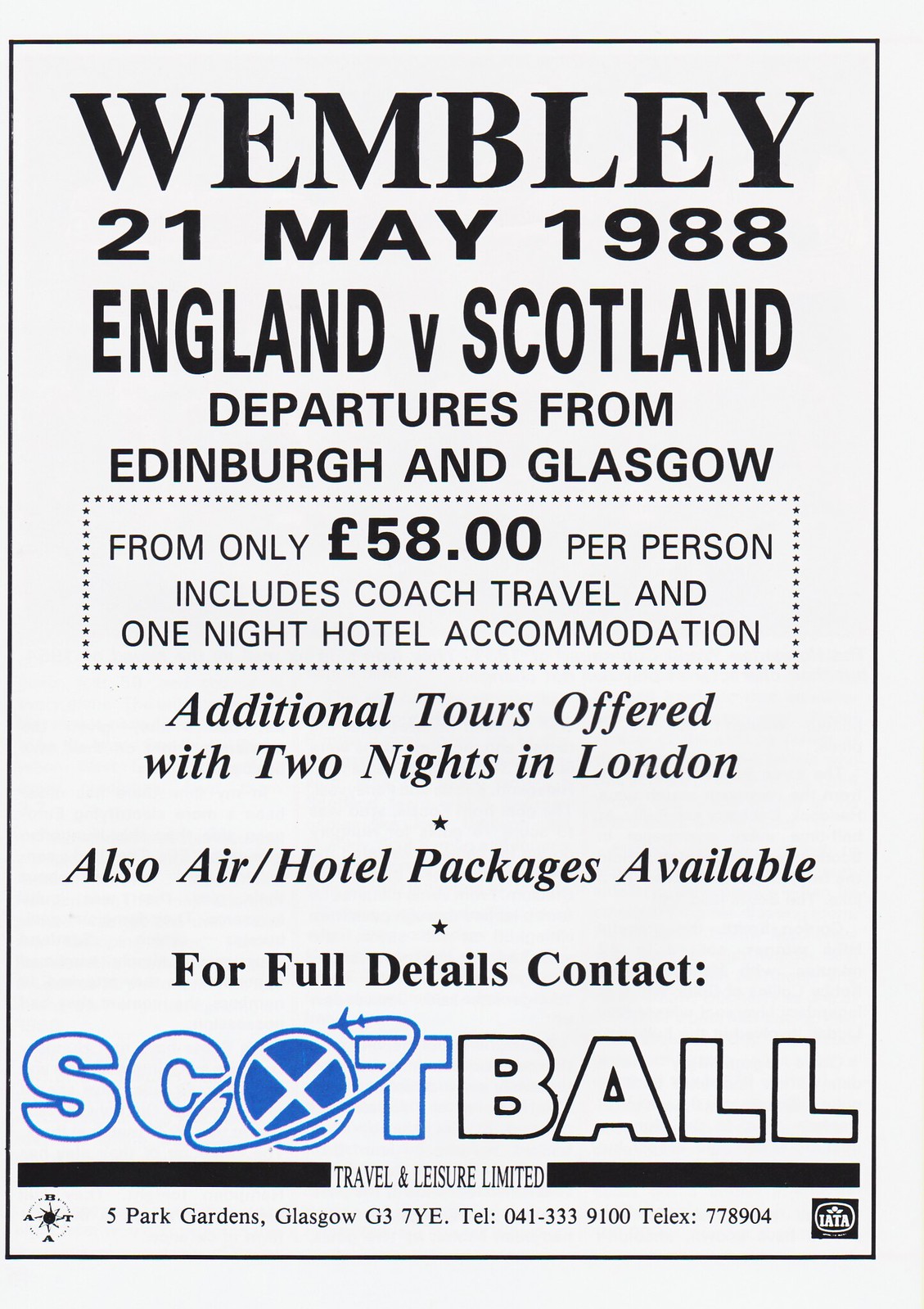The advertisement, printed on an off-white, vertically-oriented page, is predominantly black and white with certain elements in blue. Encased in a thin black border, it features various sections of text. The headline at the top reads "Wembley 21 May 1988, England vs Scotland," followed by details about departures from Edinburgh and Glasgow for only £58 per person, which includes coach travel and one-night hotel accommodation. Below this, a dotted rectangular box highlights additional offers, such as two-night tours in London, air hotel packages, and instructions for further details. Positioned prominently at the bottom is the name "Scott Ball," with "Scott" in blue and "Ball" in black, leading into the company's full title and contact details: Scott Ball Travel and Leisure Ltd, Five Park Gardens, Glasgow G37YE, telephone 041-333-9100, and Telex 778904.